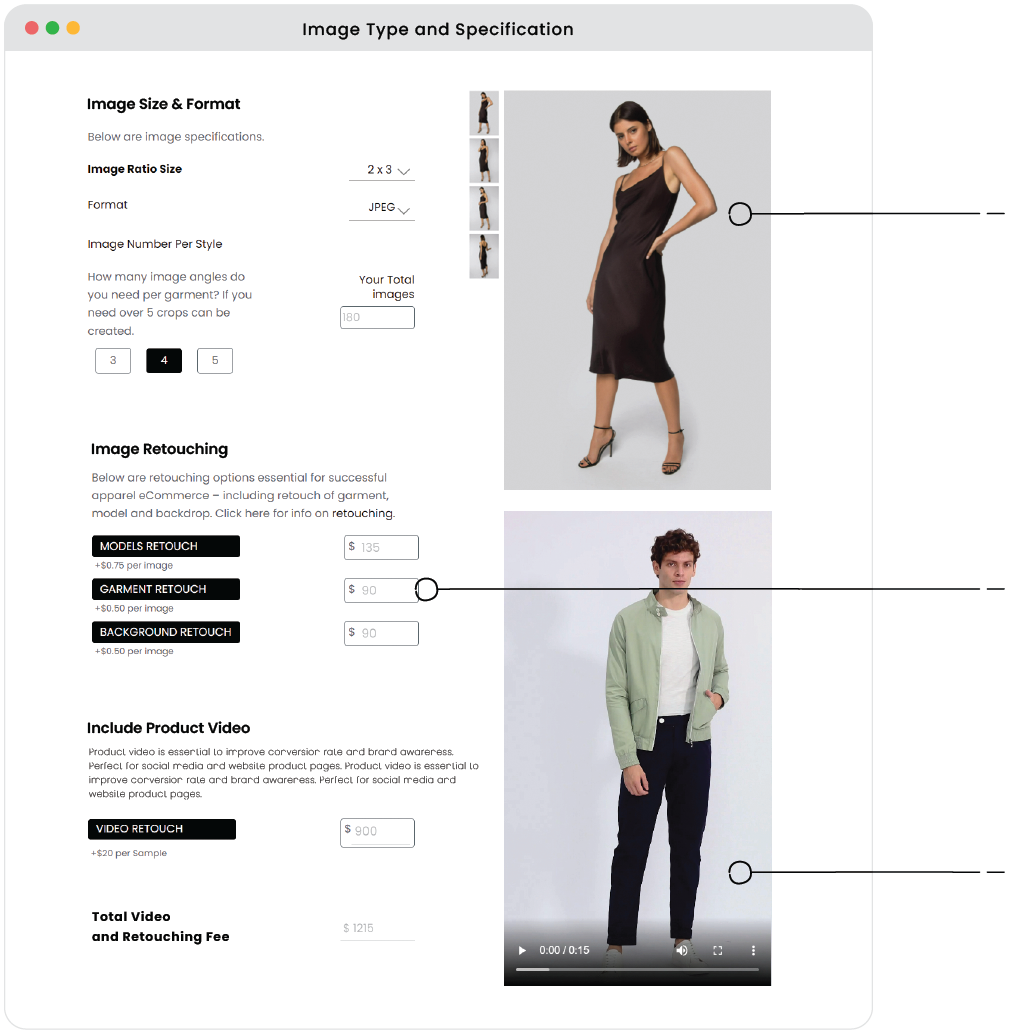**Caption:**

A screenshot of a web page captured on a Macintosh computer, identifiable by the distinctive red, yellow, and green control circles in the top left corner of the window. The web page features a horizontal gray navigation bar at the top, with "Image Type and Specification" prominently displayed in black text. The main content area, set against a clean white background, appears to be a website offering professional image and video editing services.

On the left side of the page, various options and dialog boxes are available for customizing image and video edits. These options include settings for Image Size and Format, Image Ratio Size, Image Retouching, and Include Product Video, among others, allowing users to upload and modify their media files. 

The right side of the page showcases examples of the editing capabilities. Positioned vertically, the top image features a white woman with medium-length black hair, wearing a dark red or dark brown dress and high heels, gazing directly at the camera. Below, there is another example, either an image or video, of a white man with curly brown hair, dressed in a basic white t-shirt, a green long-sleeved button-down shirt, and black slacks. These visual examples demonstrate the diverse range of editing services available on the site, from adjusting clothing and appearance to altering the overall composition of the media.